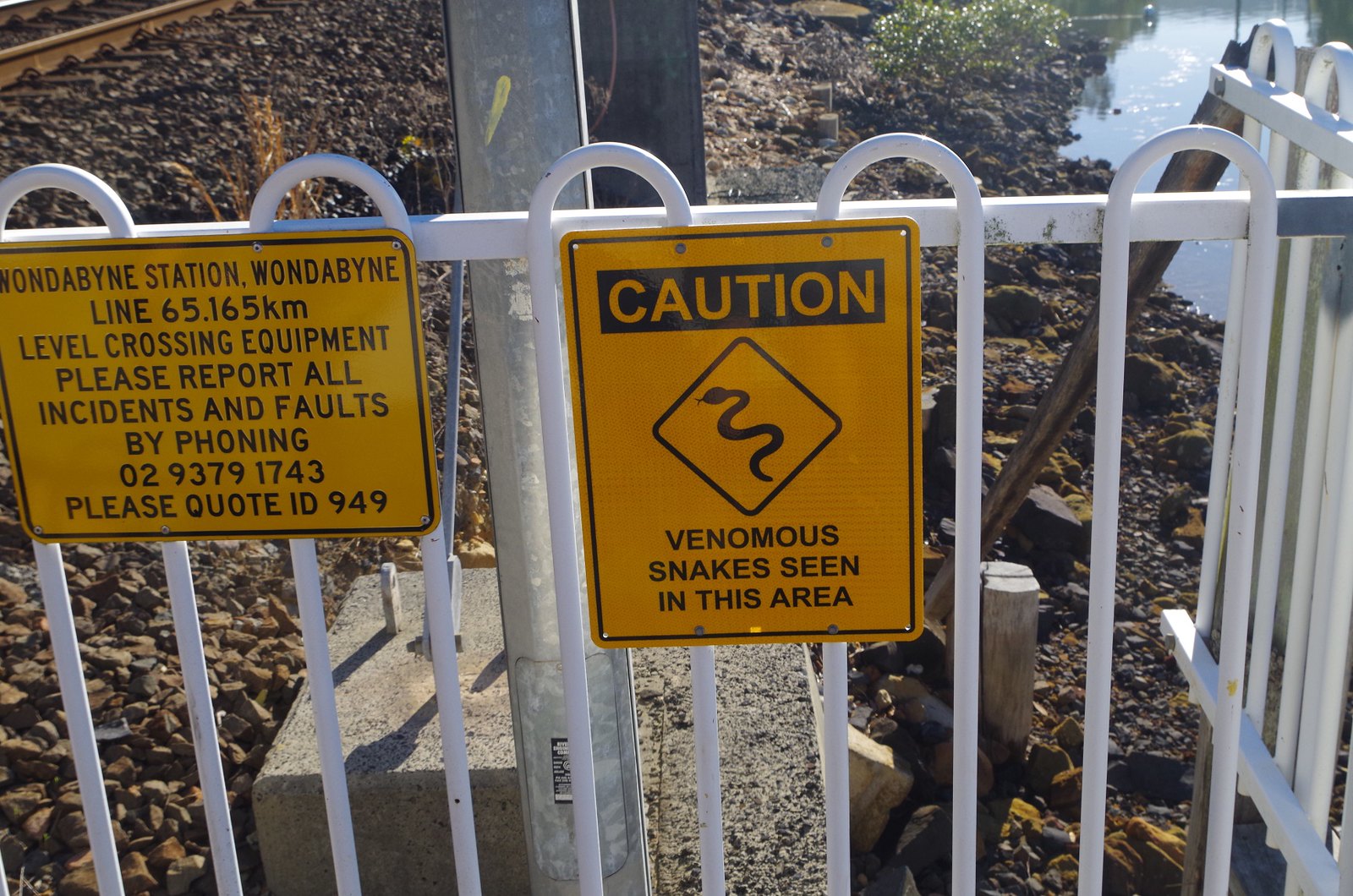In the color photograph taken outside on a bright, sunny day, the focal point is a white metal fence adorned with caution signs. The most prominent sign is in bold yellow-orange, warning "CAUTION! VENOMOUS SNAKES SEEN IN THIS AREA," and features a square diamond-shaped image with a snake illustration. To the left of this sign, another sign provides detailed information about the location, reading: "Wondabyne Station, Wondabyne Line, 65.165 kilometers, level crossing equipment, please report all incidents and faults by phoning 0293791743, please quote ID 949." Behind the fence, a range of elements are visible: to the left, dark-colored gravel surrounds train tracks, while to the right, a large mud puddle can be seen near a body of water with a muddy, rocky shore. Taller in the background, a metal pole and possibly an I-beam appear to be part of an industrial setup, slightly dilapidated. The curved vertical posts of the fence and a concrete pillar, seemingly a light post, add to the detailed landscape captured in this scene.